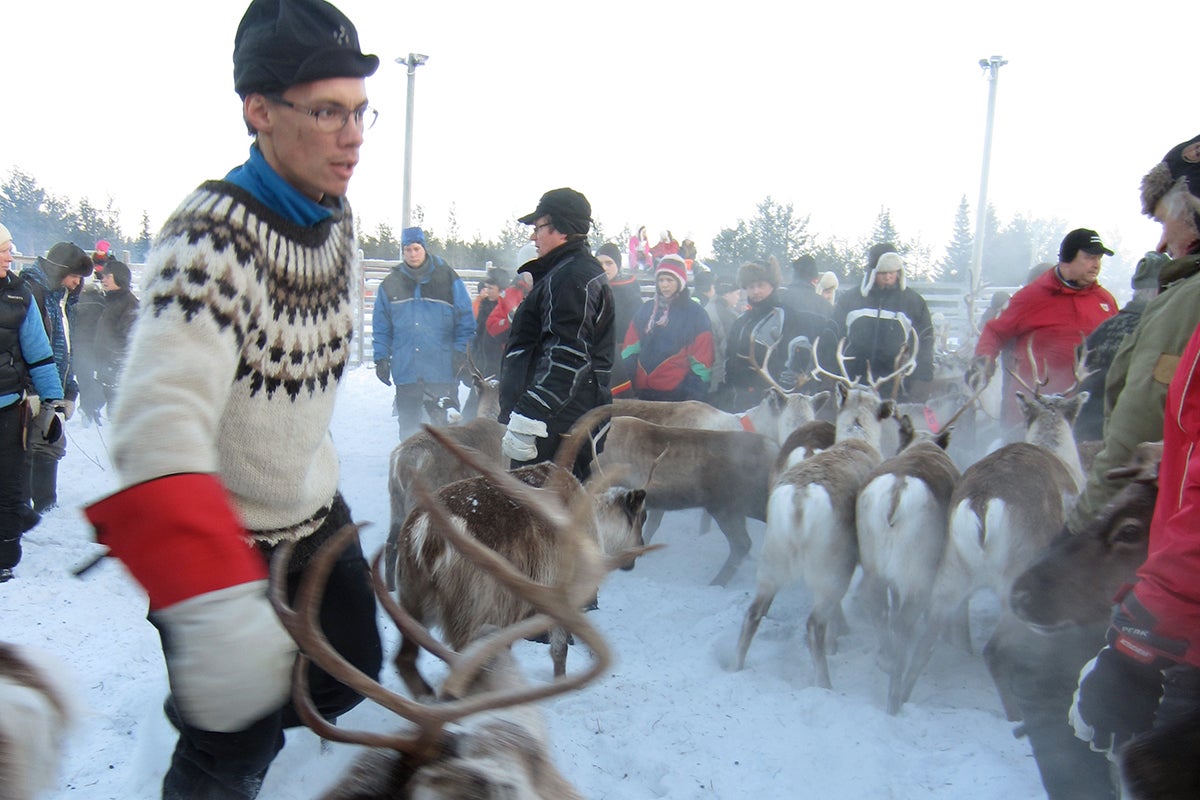In this digital wintertime photo, a snowy or cloudy landscape forms the backdrop, featuring a tree line of green pine trees. The foreground showcases a group of people dressed in various winter clothes, standing in a circle. Two gentlemen are the main focus: the one on the left, a Caucasian male, sports glasses, a black hat, a white sweater with a red design over a blue turtleneck, and oversized red-and-gray gloves. The gentleman on the right, positioned slightly farther back, wears a black heavy jacket with gray stripes, a fancier black baseball hat, white gloves, and glasses. Amidst the people are seven or eight small-statured reindeer with pointy horns, some facing away with brown tops and white legs. Everyone, including the reindeer, has visible breath vapor due to the cold air. The scene is slightly hazy or foggy, enhancing the wintry atmosphere, and some tall structures resembling cell towers are visible in the background.